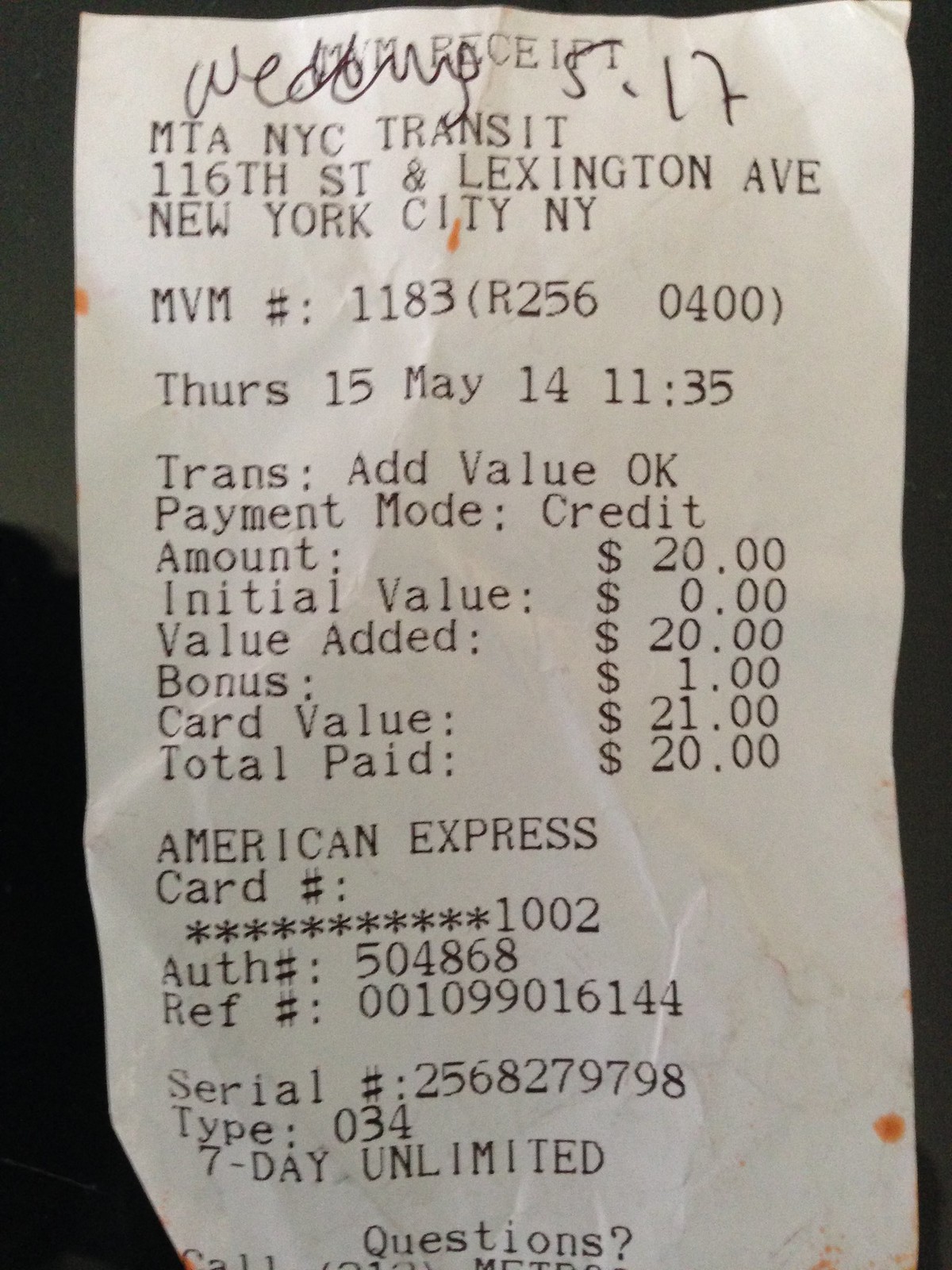This photograph captures a crumpled receipt from MTA New York City Transit, prominently displayed against a predominantly black background, with the top left quarter exhibiting a dark gray hue that suggests a nearby light source. The lighting angle from the top left is evident from the reflections and shadows on the creased receipt. The receipt details a purchase amount of $20 paid with an American Express card, specifically for a seven-day unlimited ticket, presumably for the NYC subway system. The issuing location is identified as 116th Street and Lexington Avenue, New York City, New York. The transaction occurred on Thursday, May 15th, documenting the date of purchase for this transit pass.